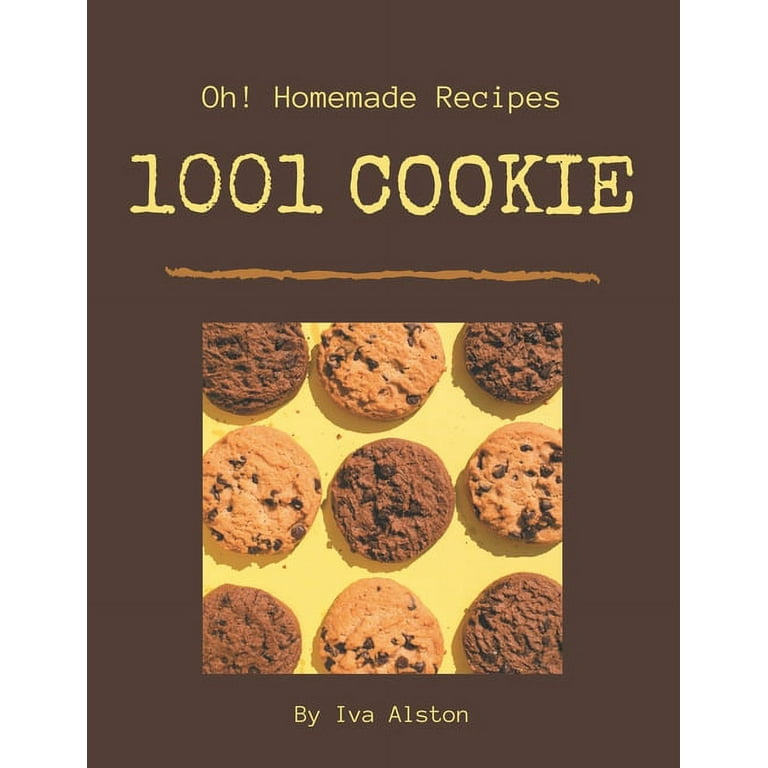The image is a vertically aligned rectangular picture resembling a cookbook cover with a dark brown background and no border. At the top, the title reads "O! Homemade Recipes," with an exclamation mark, in yellow text. Below the title, centered in larger all-caps yellow letters, it says "1,001 Cookie," with a light brown hand-drawn line beneath it. The bottom part of the cover features a square section with a yellow background resembling a table, displaying nine cookies in three rows of three. The cookies alternate in appearance: darker brown chocolate chocolate chip cookies and lighter chocolate chip cookies. The top row has a chocolate cookie, a chocolate chip cookie, and a chocolate chocolate chip cookie; the middle row shows two chocolate chip cookies on the sides and a chocolate chocolate chip cookie in the center; the bottom row includes a chocolate chocolate chip cookie, a chocolate chip cookie, and another chocolate chocolate chip cookie. At the very bottom, the author's name, "By Ivor Alston," is written in yellow letters.